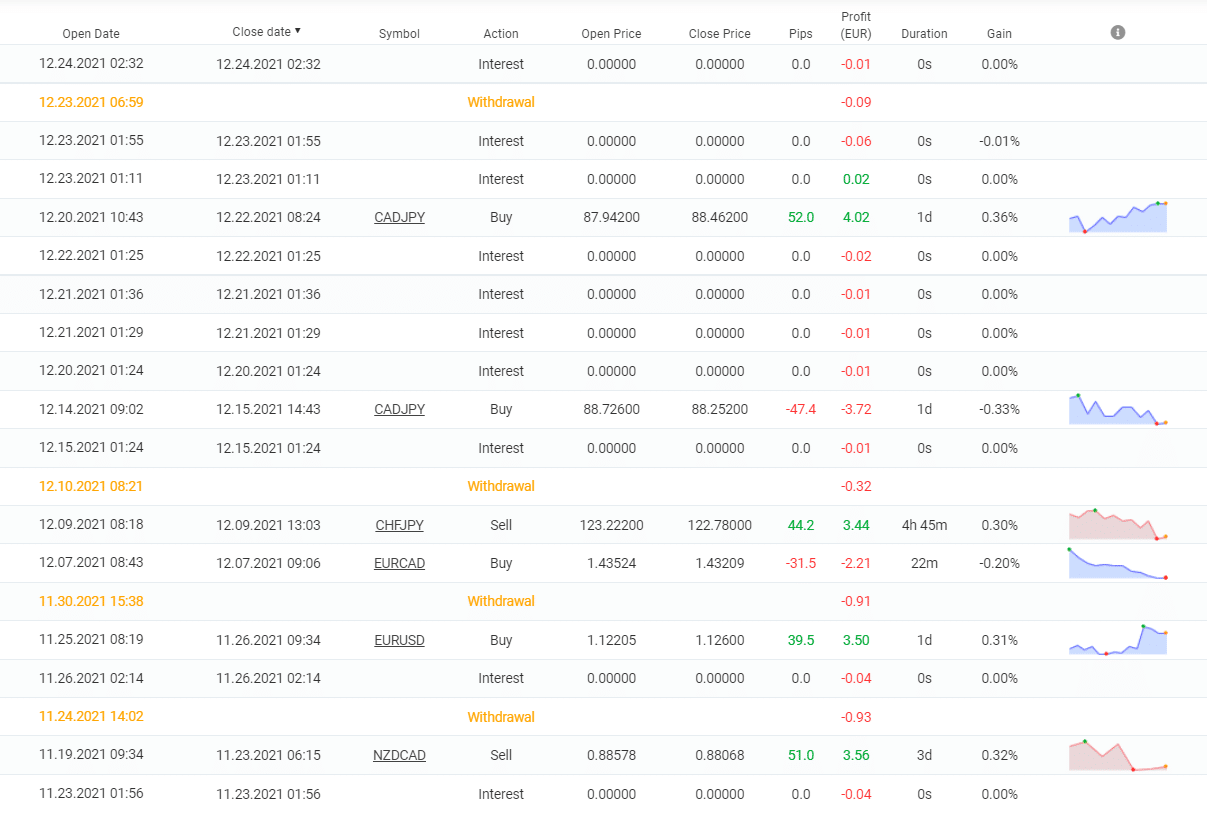The image depicts a comprehensive table tracking various stock market investments. The table contains multiple columns labeled as: "Open Date," "Close Date," "Symbol," "Action," "Open Price," "Close Price," "Pips," "Profit" (denoted in euros), "Duration," and "Gain." Each row of the table represents an individual trade, with data captured for each respective category.

At the top of the table, the most recent entry is dated December 24th. The entries are organized in descending order, with the earliest date listed at the bottom. For instance, the entry at the bottom is dated November 23, 2021, with an open time of 1:56 and a close time of 1:56 on the same day.

Each row provides detailed information about the trades, such as the stock symbol, the type of action (e.g., buy or sell), the prices at which stocks were opened and closed, the number of pips gained or lost, the profit in euros, the duration of the trade, and the overall gain percentage.

Some rows also feature small graphs, displayed in either blue or red, providing a visual representation of the trade performance. The color and pattern of these graphs vary, indicating different market outcomes for each trade.